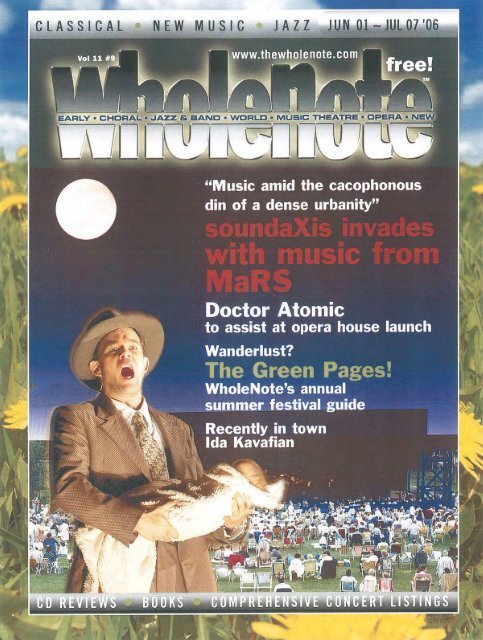This image is a detailed photographic advertisement for a publication or event, possibly the front cover of a magazine named "Whole Note." The layout features a prominent banner across the top with text in a gray background that reads "Classical New Music Jazz, June 1st to July 7th, 2006." In the upper left corner, it states "Volume 11, Number 9," with the website "www.thewholenote.com" above it. To the right, in bold, it says "Free."

Central to the image is a striking photograph of a man in a 1950s-style brown three-piece suit, wide-brimmed hat, and tie. His mouth is open, suggesting he is singing. He holds a swaddled baby, just the top of the head visible. Above him, there's a moon in a dark sky, adding to the atmospheric setting. Below, an audience is seated in lawn chairs, watching what seems to be a performance. The background is adorned with flowers and hints at a blue sky, merging the urban with the natural.

Text overlays include "Early Cultural Jazz Band World Music Theater Opera New" in a bold banner across the word "Whole Note." Additional intriguing phrases such as "Music amid the cacophonous din of a dense urbanity" and "Sound Access invades with music from Mars - Dr. Atomic to assist at opera house launch" are scattered, hinting at the eclectic and vibrant content featured in the publication.